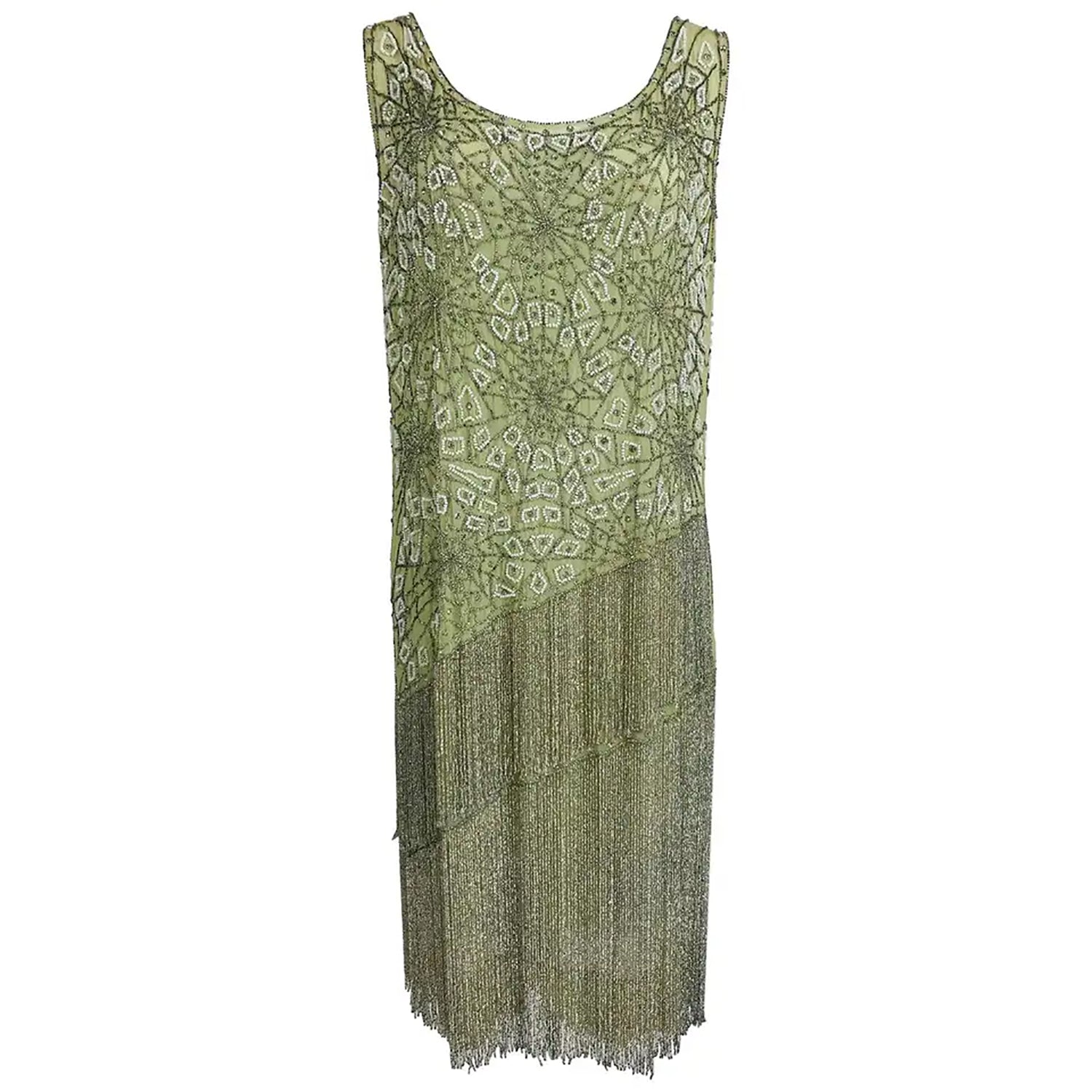The image displays an elegant, vintage-style green dress with intricate detailing. The sleeveless dress features a broad, arched neckline without cuffs, reminiscent of 1920s flapper fashion. The upper part of the dress is adorned with delicate green spiderweb-like patterns interspersed with white tiny bead embroidery, creating a visually captivating design. Thin straps gracefully extend from the shoulders, forming the structure of the dress. As the pattern descends towards the waist, it transitions into diagonal lines, giving way to a section of the dress adorned with green lace. The lace, a darker shade of green, is decorated with strict line patterns and has a second layer visible behind it. This lace section extends nearly to the knees, interwoven with grayish-green threads that maintain the dress's elegant flow. The background of the image is a plain white, placing full emphasis on the dress's intricate details and overall design.